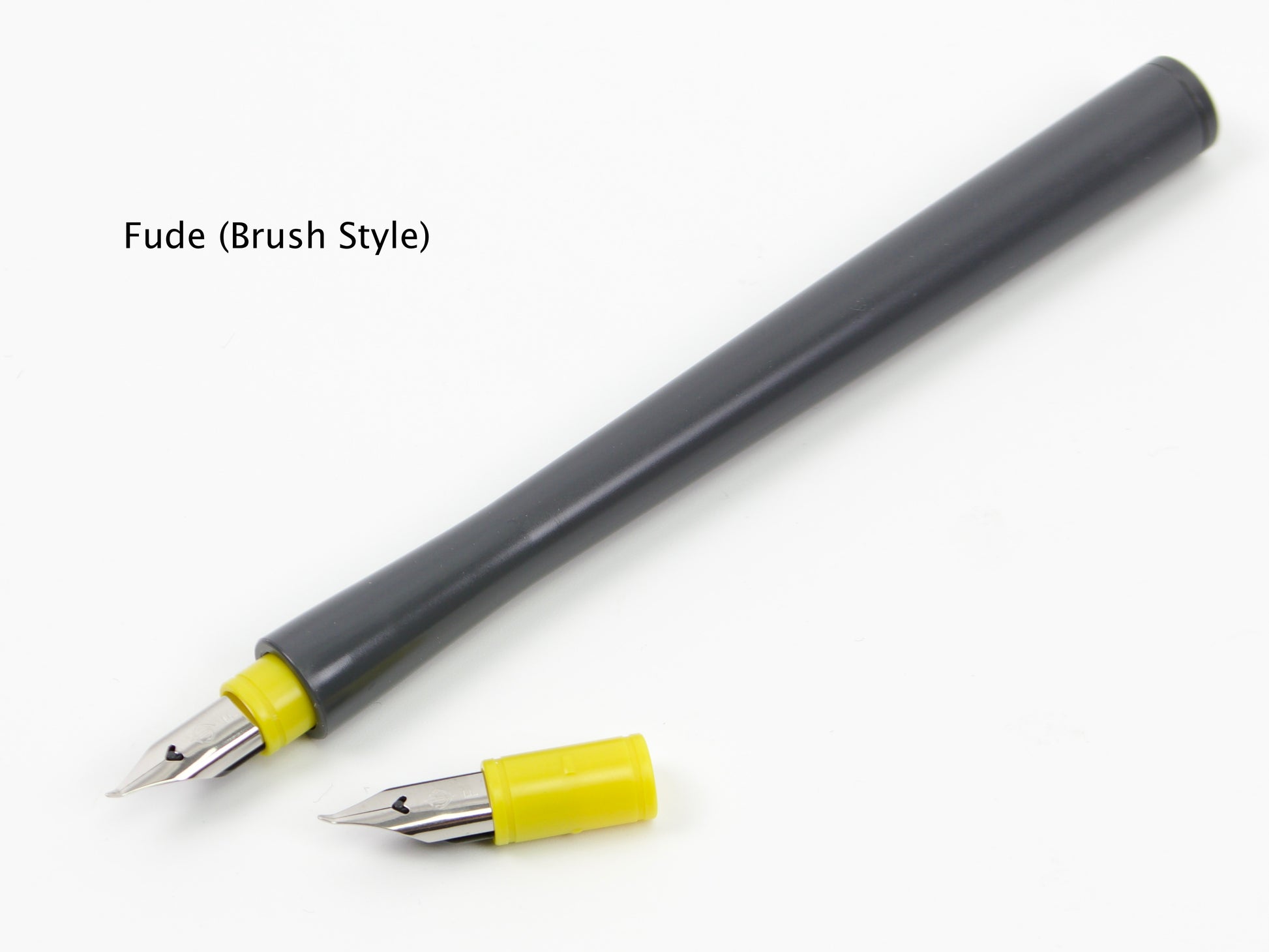The image displays a black fountain pen on a white background. The pen, labeled "Fude (brush style)" in black text located in the top left corner of the image, features two tips. The main body of the pen starts from the top right corner and extends diagonally toward the lower left. The pen narrows just before reaching the tip, where it widens again, ending in a bright silver, sharply pointed nib with a small heart-shaped indentation near the tip. The pen has a distinctive yellow plastic section near the tip, which is designed to secure the nib. An additional silver nib, also with a yellow plastic holder, is placed next to the pen, suggesting interchangeable tips for different writing styles.